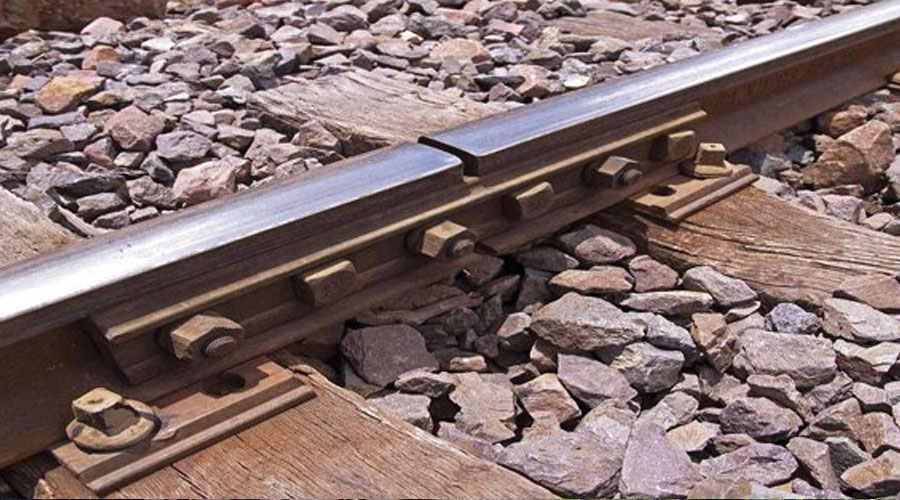This close-up photograph captures the intricate details of a railroad track, showcasing the connection point where two steel tracks meet, secured by a metal plate with six large rusted bolts and nuts. The tracks are held in place by weathered wooden railroad ties, which display signs of aging and sun-bleached patina. Between these ties lies a bed of gravel composed of small to medium-sized rocks in hues of gray and rusty red. Despite the age-worn appearance of the wood and the rust on the bolts, the metal tracks themselves are smooth and gleaming, indicating recent maintenance or heavy use. The image stretches from left to right, emphasizing a single track that is meticulously maintained but surrounded by natural elements that have visibly withstood the test of time.